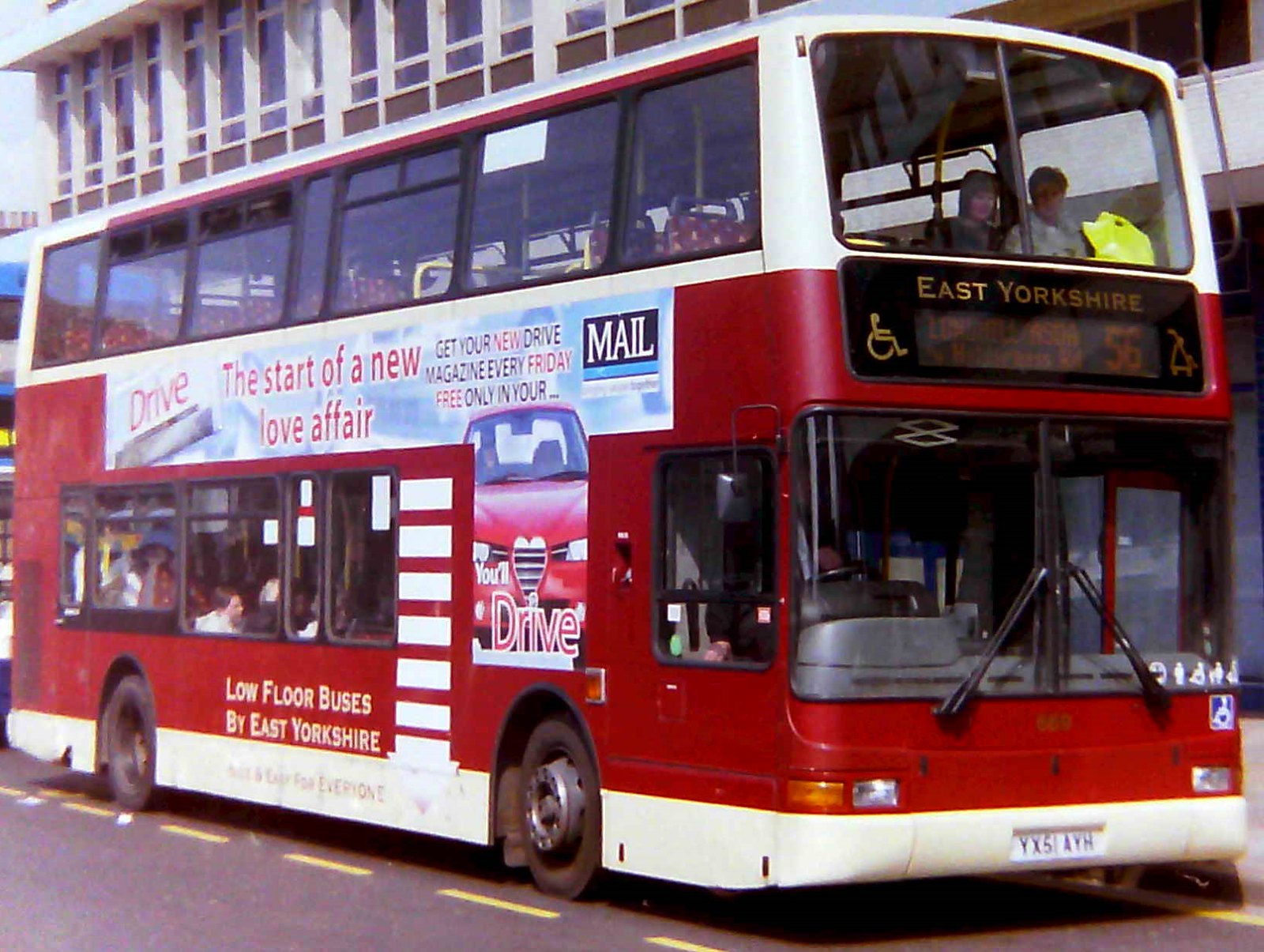This image depicts a red double-decker bus, identified as an East Yorkshire service. The bus is parked at a curb, facing towards the right of the frame, with its back end slanting towards the middle left. Prominently displayed on the front of the bus is the text "East Yorkshire" in yellow on a black background, alongside an LED display and a symbol indicating wheelchair accessibility. The destination label reads "Bus 56."

The side of the bus features a white and blue banner advertising "Drive, the start of a new love affair" in red font. The advertisement encourages readers to get their free New Drive magazine every Friday, exclusively available in Europe, and includes an image of a red car with the phrase "you'll drive." Adjacent to this, in white lettering on a blue background, is the word "MAIL." Below the windows of the lower level, it reads "Low Floor Buses by East Yorkshire" in white text against the red of the bus.

The bus is equipped with numerous windows on both the lower and upper decks, through which passengers can be seen. This particular scene appears to be set in London, evidenced by the street and urban surroundings, including a three-story building visible behind the bus. The license plate is also visible at the front of the bus.